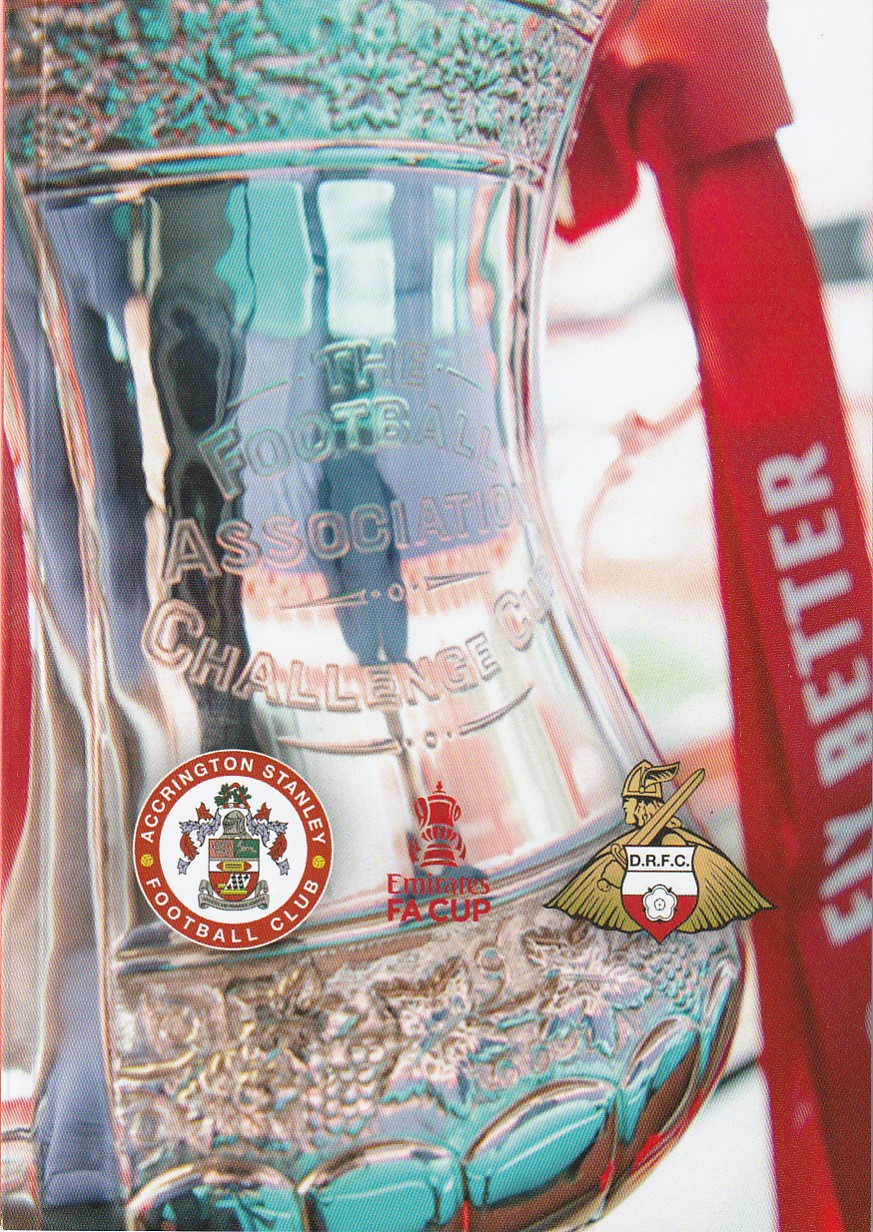The image is a detailed close-up of a shiny, reflective trophy, specifically the Football Association Challenge Cup. The trophy is partially shown, but it's clear that it flares out at the top and bottom, with intricate floral engravings adorning these sections. There are green, blue, purple, pink, and reddish hues reflecting off its polished surface, adding to its visual appeal. The inscription "Football Association Challenge Cup" is clearly visible. Three logos are overlaid on the image: 

On the left, the emblem of Accrington Stanley Football Club is featured, with a detailed coat of arms encased in a red circular border. 

In the center, there’s the Emirates FA Cup logo in red, consisting of a stylized simplistic cup and the text "Emirates FA Cup" beneath it. There is also a red ribbon with "Fly Better" written in white along the side. 

On the right, a golden, bronze-colored insignia depicts a soldier with a sword and a Viking-like helmet, accompanied by a shield with the initials DRFC, divided into white and red fields with a floral pattern at the center.

Each of these elements contributes to the rich and elaborate design of the photograph, highlighting the prestigious nature of the championship trophy.